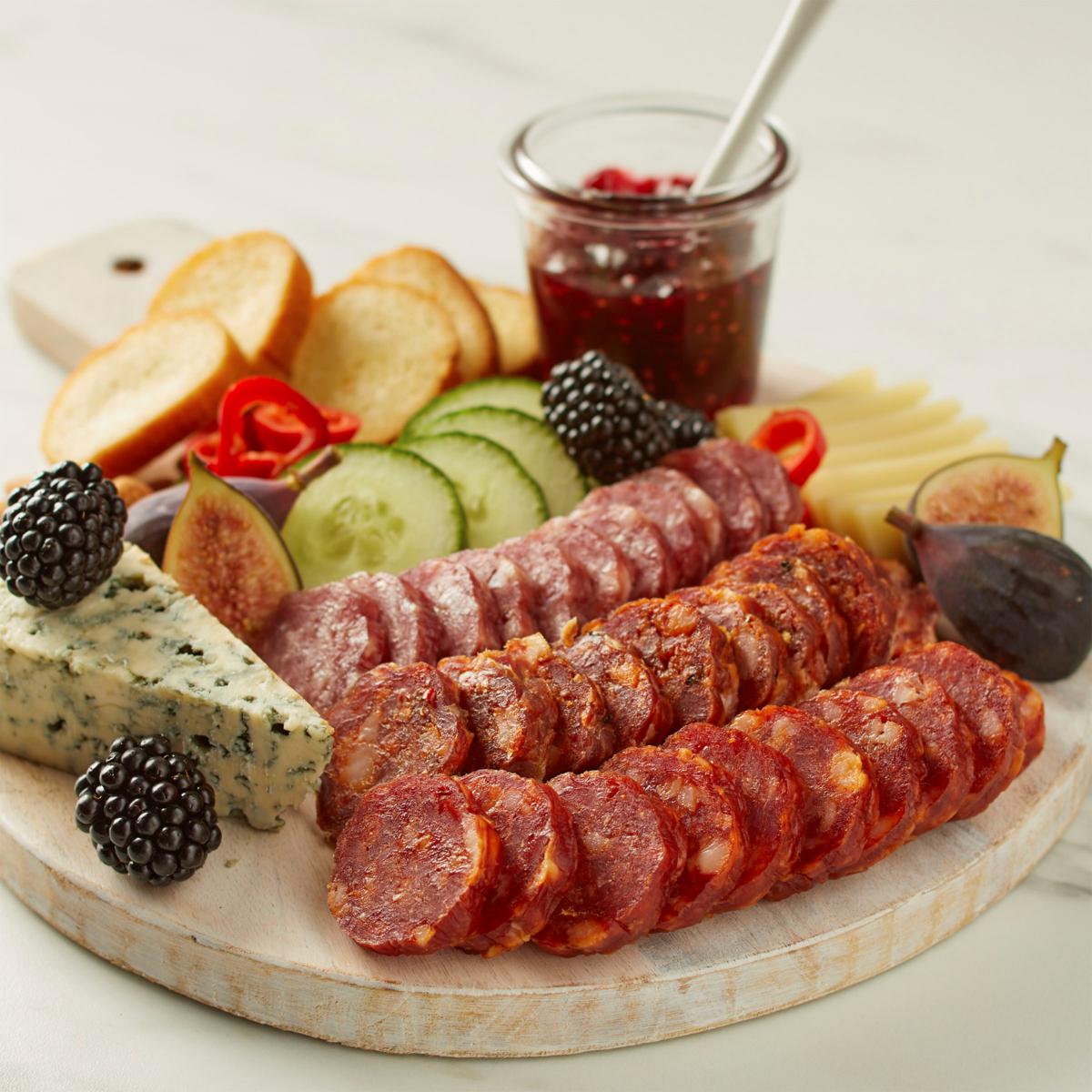This image features a meticulously arranged charcuterie board set on a light brown, circular wooden platter, possibly with a distressed and painted finish. The board displays an array of appetizers ideal for snacking or entertaining. Prominently in the foreground, there are three rows of sliced meats, likely pepperoni or salami. Adjacent to the meats on the left rests a wedge of blue cheese, topped by a blackberry, with several other blackberries scattered across the platter.

A small glass jar of red jam or raspberry preserves, complete with a spoon, is positioned towards the rear of the board. Surrounding the meats are rows of cucumber slices, apples, or perhaps more types of cheese. Additional elements include round cuts of bread or bagel crisps and slices of figs, both whole and halved, revealing their centers.

Pepper slices and some other unidentified food items add to the colorful spread. The board appears to have a handle with a hanging hole, attesting to its practicality and aesthetic appeal. The charcuterie board is set against a light tan background, enhancing the visual presentation of the assorted delicacies.